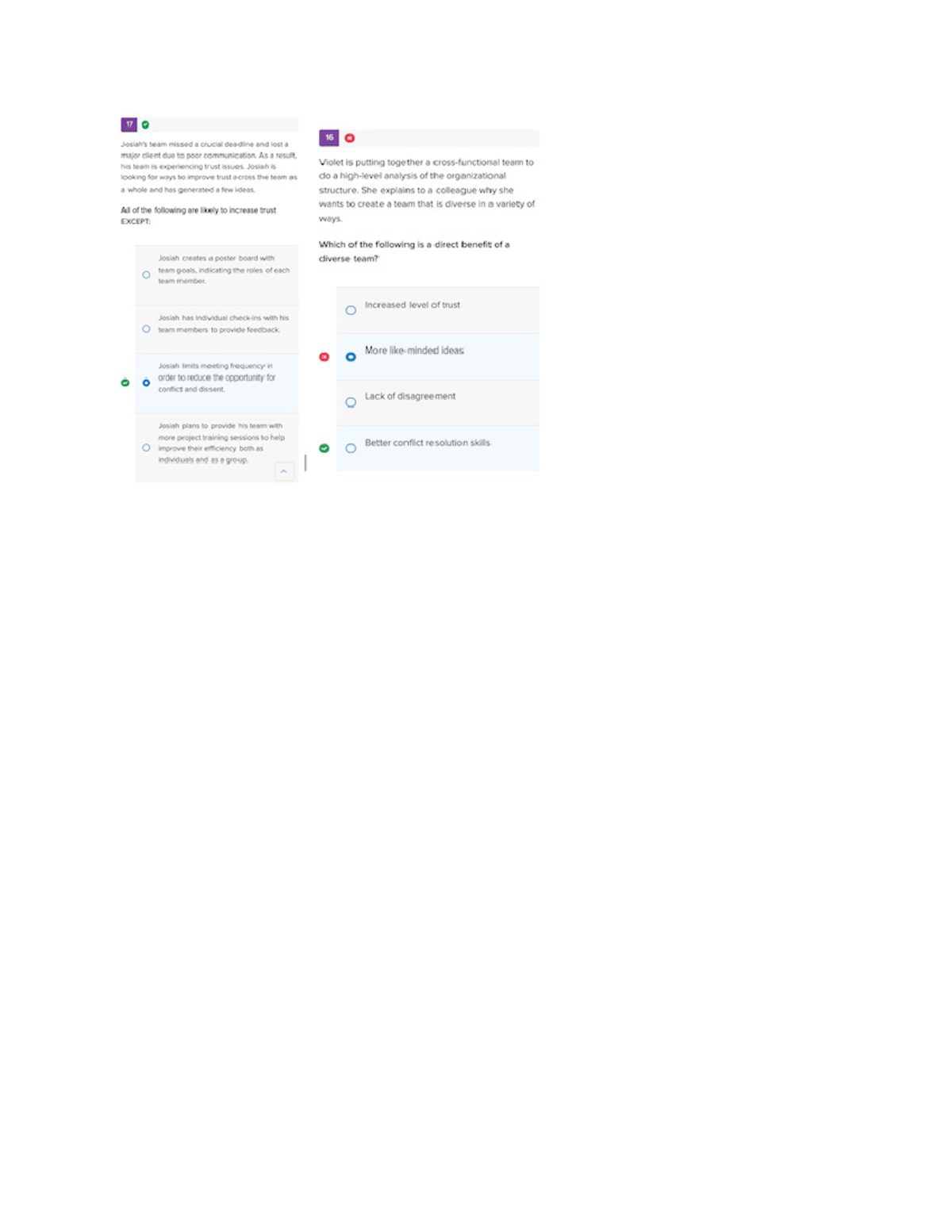A miniature screenshot appears to capture a segment of a quiz interface. In the top left corner, there is a dark purple square containing the numerical indicators of the questions. To the left, it displays the number "17" accompanied by a green circle with a white checkmark, suggesting a correct answer for that question. Adjacent to this, the number "16" is shown next to a red circle featuring a white 'X', signifying an incorrect answer for the corresponding question. Although the exact questions for both items are not visible, a portion of the follow-up question for item 16 can be discerned, asking, "Which of the following is a direct benefit of a diverse team?"